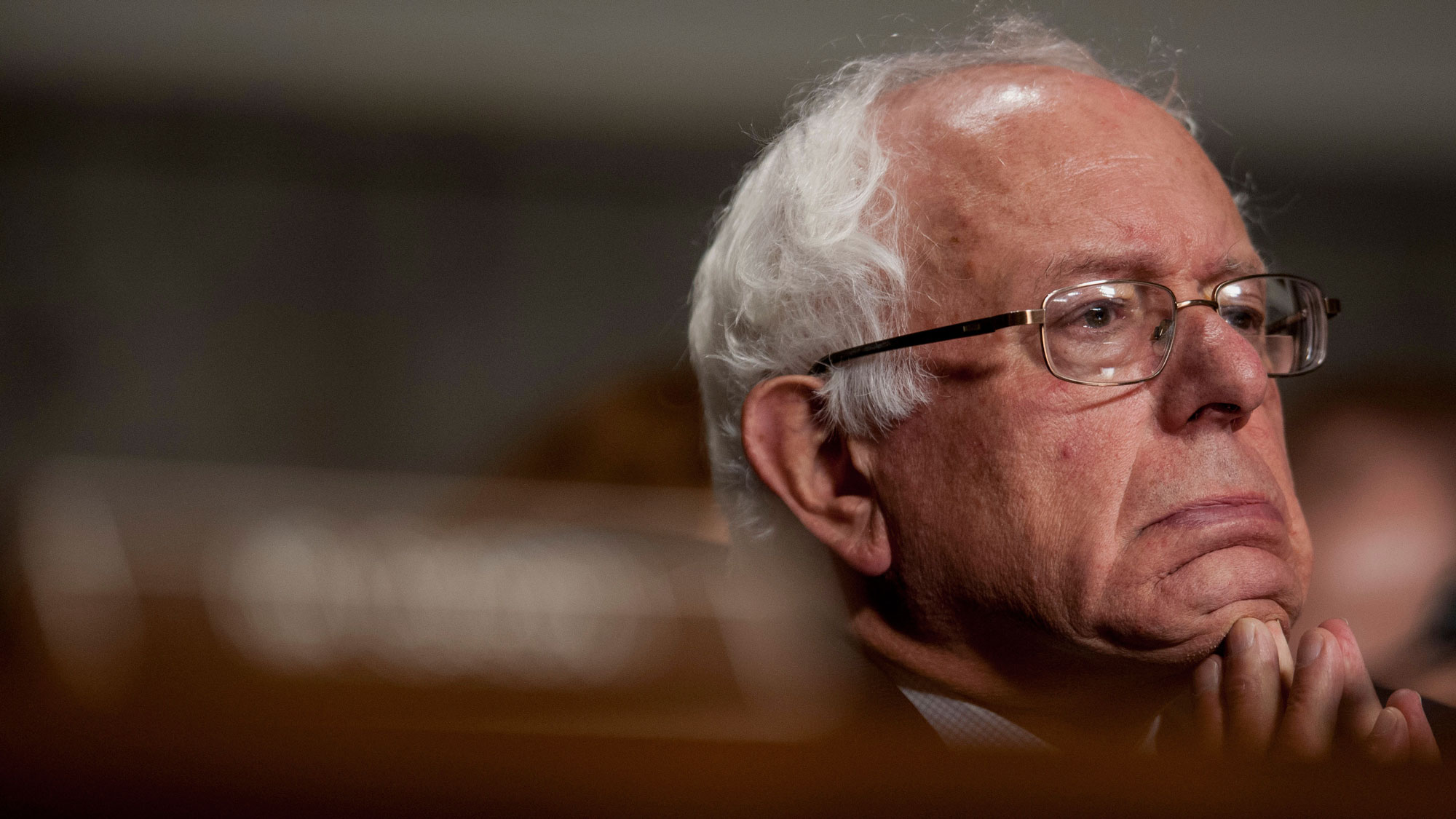In the image, an older gentleman with gray hair, possibly Bernie Sanders or Warren Buffett, is deeply engrossed in thought. He has a solemn expression, with furrowed brows and a slight scowl, indicative of intense focus or mild frustration. The man is wearing glasses with rounded, rectangular frames and rests his chin on his interlaced fingertips in a contemplative pose. His white collar suggests he might be wearing a suit. The background is blurred, with an indistinct shadowy box next to him, adding to the image's overall pensive mood. The angle is not quite a profile but captures him from a diagonal perspective, highlighting his serious demeanor.